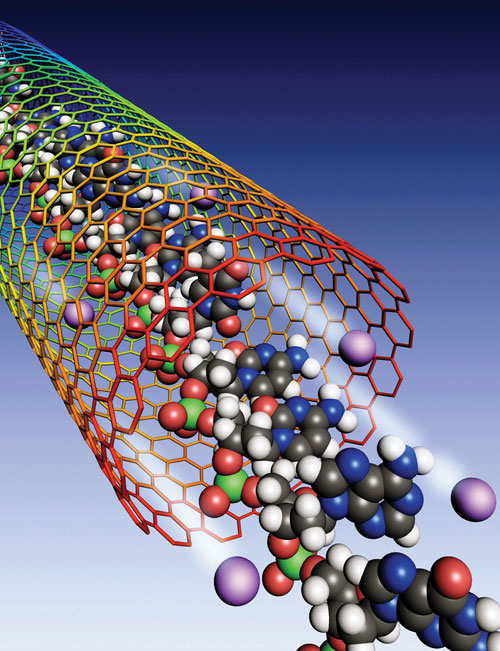This image is a digitally created graphic featuring a vibrant, complex design. The background gradient starts with a dark blue at the top, which fades into lighter shades and eventually turns white towards the bottom. Central to the image is a basket-like structure situated in the top left, positioned to the center, seemingly pouring out various colorful balls. These spheres are part of a detailed computer rendering, possibly symbolizing molecules or atoms, arranged in distinct patterns.

The main focal point is a cylindrical shape made of interlocking rods that form hexagons, resembling a curled-up chain-link fence. This cylinder transitions through a vibrant spectrum beginning with red at the open end closest to the viewer, then blending into orange, yellow, green, and finally blue. Inside this cylindrical structure, the spheres are connected in intricate patterns typical of molecular diagrams. The colors of these spheres span different shades of blue, purple, green, yellow, orange, red, gray, and white, with many joined together primarily by gray spheres. The overall visual suggests it could be a digital graphic often used in a healthcare setting, emphasizing a scientifically inspired, abstract representation.